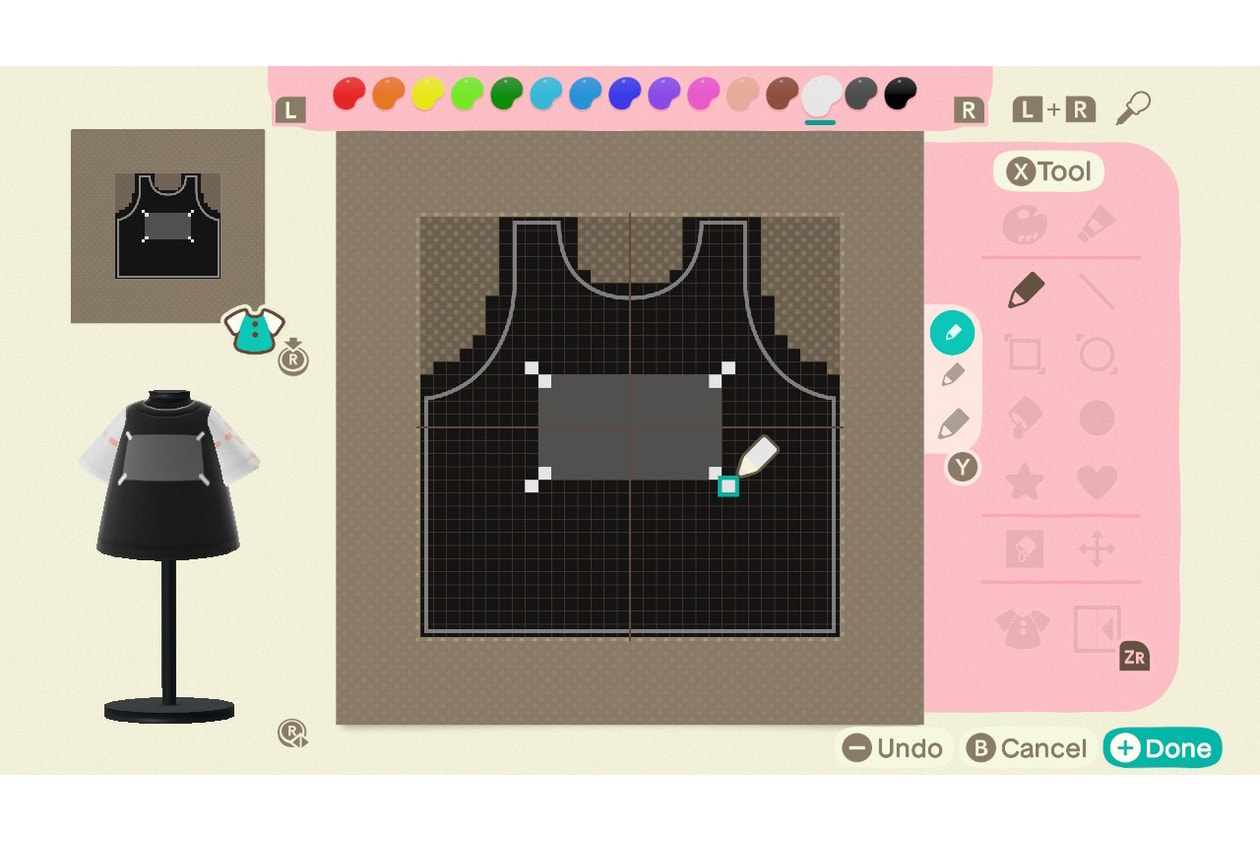The image is a detailed color screenshot of a graphic editing or sewing pattern layout program in landscape orientation. Central to the screenshot is a black outline of a tank top with a gray horizontal rectangle across the chest area, positioned against a brown checkered mat. The tank top template serves as a workspace for users to draw and edit artwork. 

Above the tank top template is a painter's palette featuring a spectrum of colors, ranging from red through black, encompassing every shade of the rainbow. The color white is currently selected. On the right-hand side of the screen, there is a vertical tool navigation panel with dual rows of icons for various graphic editing functions, including tools for cropping, drawing (pencil and pen), shaping (stars and hearts), and line creation. Additional navigation buttons, such as undo, cancel, and completion options, are located at the bottom.

To the lower left of the main template, there's a mannequin stand with a shirt model displaying an identical pattern—a black tank top with white short sleeves and a gray rectangle on the chest—positioned against another slightly larger brown mat. Above this is a preview section showcasing variations of the central template, including a small shirt illustration with aqua fabric and white leaves. This intricate layout, set against a cream-colored background, highlights the program's comprehensive design and editing tools.